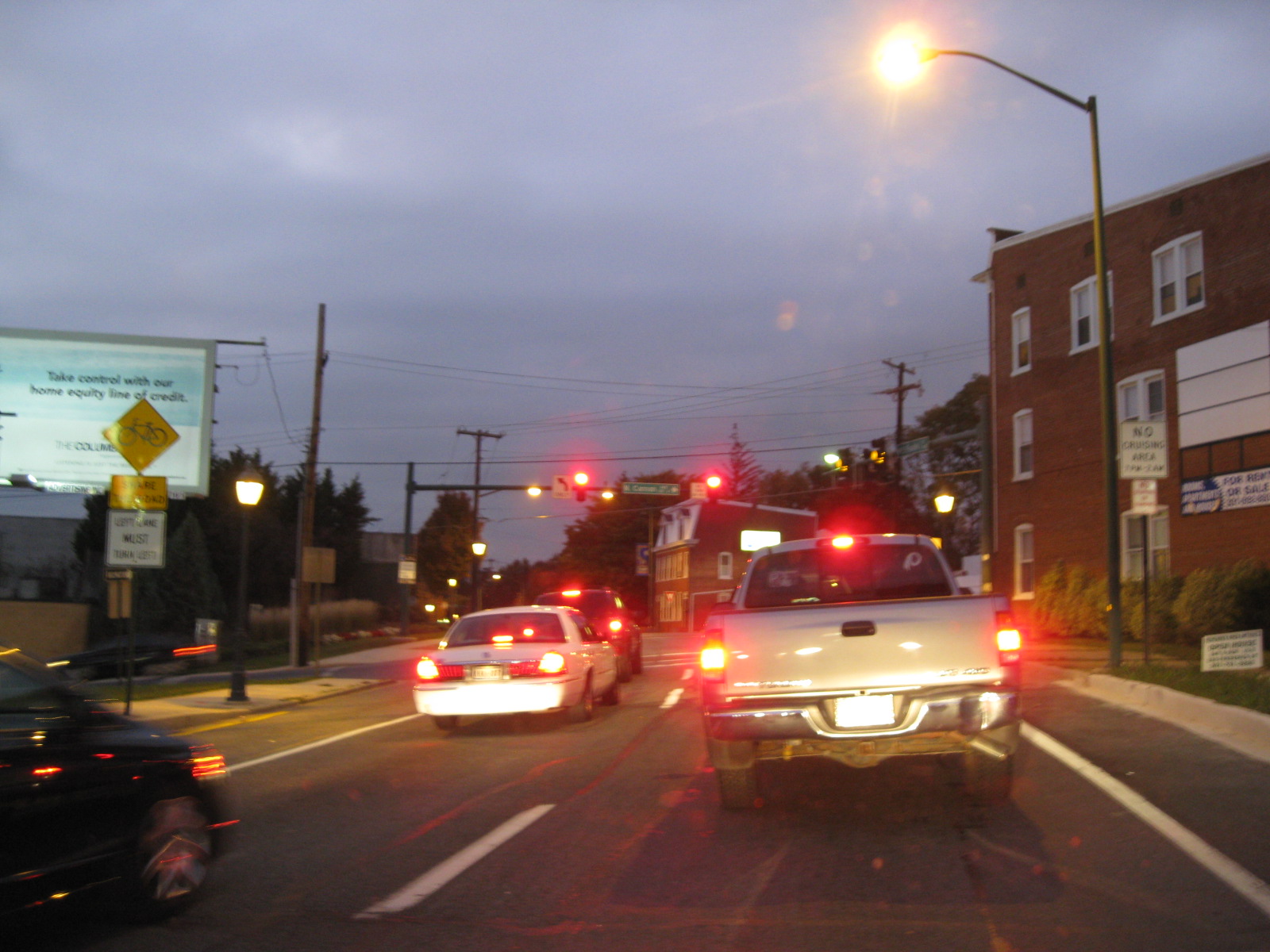This detailed nighttime photograph captures a street from the perspective of a car stopped in the right lane, likely taken from a dash cam. In front of the car is a white pickup truck with its brake lights on, while the left lane contains a white sedan, a red truck, and a black car. All vehicles are halted at a red light at a busy intersection. The scene is well-illuminated by various streetlights, and traffic signals hang overhead, casting a twilight glow under the cloudy sky. On the right stands a three-story brown brick building with several windows, and on the left, multiple traffic signs are visible, including a bicycle crossing sign and a left-turn-only sign. A billboard reading "Take control with our home equity line of credit" looms above, accompanied by power poles and their crisscrossing lines. The meticulous layout of lane markings and the assortment of urban elements, such as an old-fashioned pedestrian street lamp and various traffic signs, enhance the urban atmosphere of the scene.